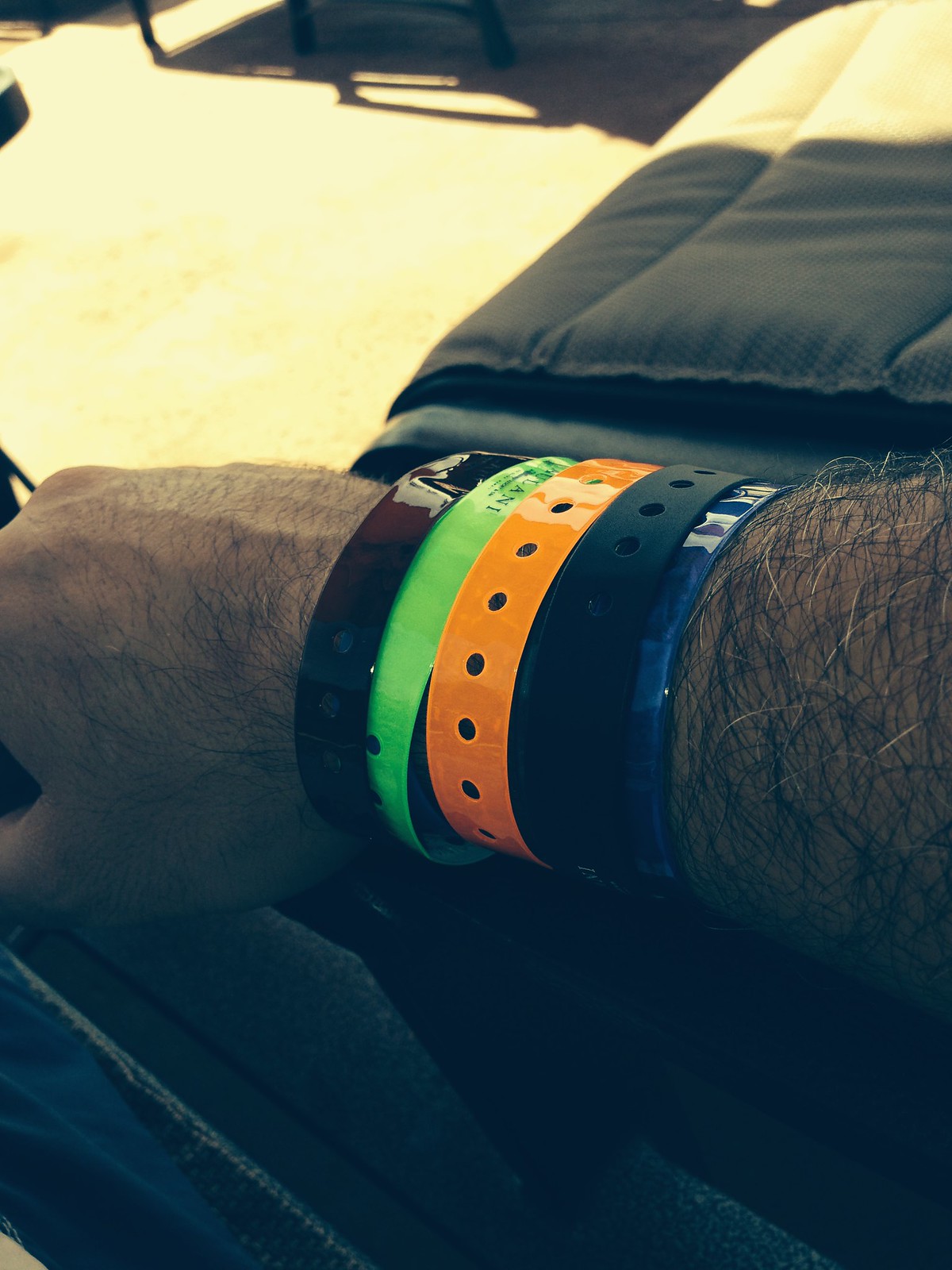The close-up image captures the forearm and hand of a man with tanned, Caucasian skin, heavily adorned with various wristbands. His arm, featuring a mix of dark and gray coarse hair, is prominently displayed from the knuckles to just below the elbow. The numerous wristbands, some made of plastic and others appearing to be leather, are detailed in color: a dark brown, lime green with writing, shiny orange, black leather, and blue with white writing or light reflection. His hand is closed in a slight fist. Above the arm appears to be a two-toned comforter or blanket, half black and half off-white, resting on a black surface. The background is generally off-white with hints of black, possibly from a seat, suggesting the setting might be outside or in a vehicle.